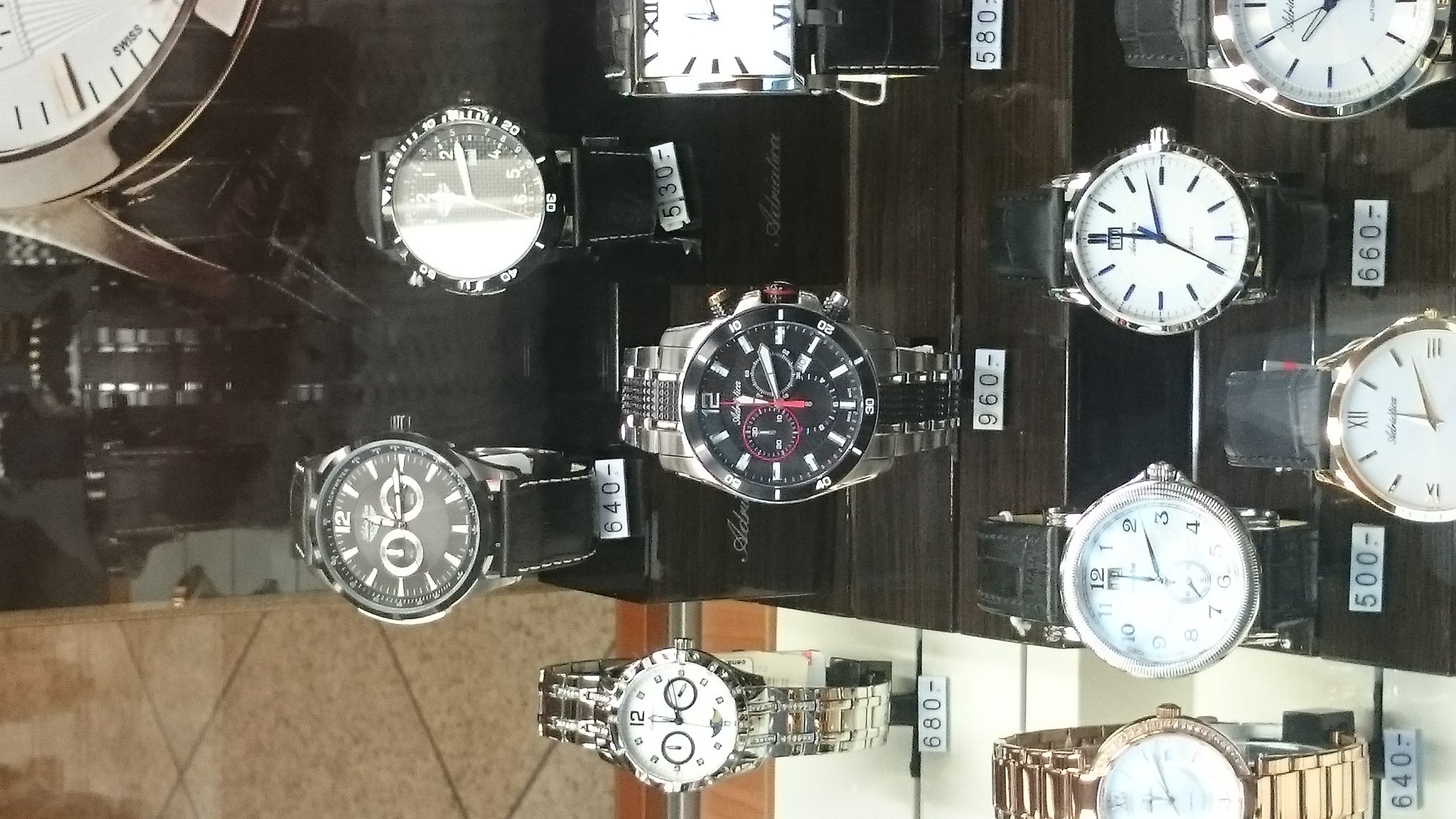This image is a meticulously detailed, bird's eye view photograph of a display case filled with various watches, presented in a landscape format. The reflection on the left side of the image suggests a glass panel protecting the timepieces beneath. However, the orientation of the photo appears to be rotated 90 degrees clockwise, implying that it was originally taken in portrait mode. The display showcases an array of watches, each positioned with price tags visible. The topmost watches are priced at $640, $530, and others even reaching up to $960, though the currency is not specified.